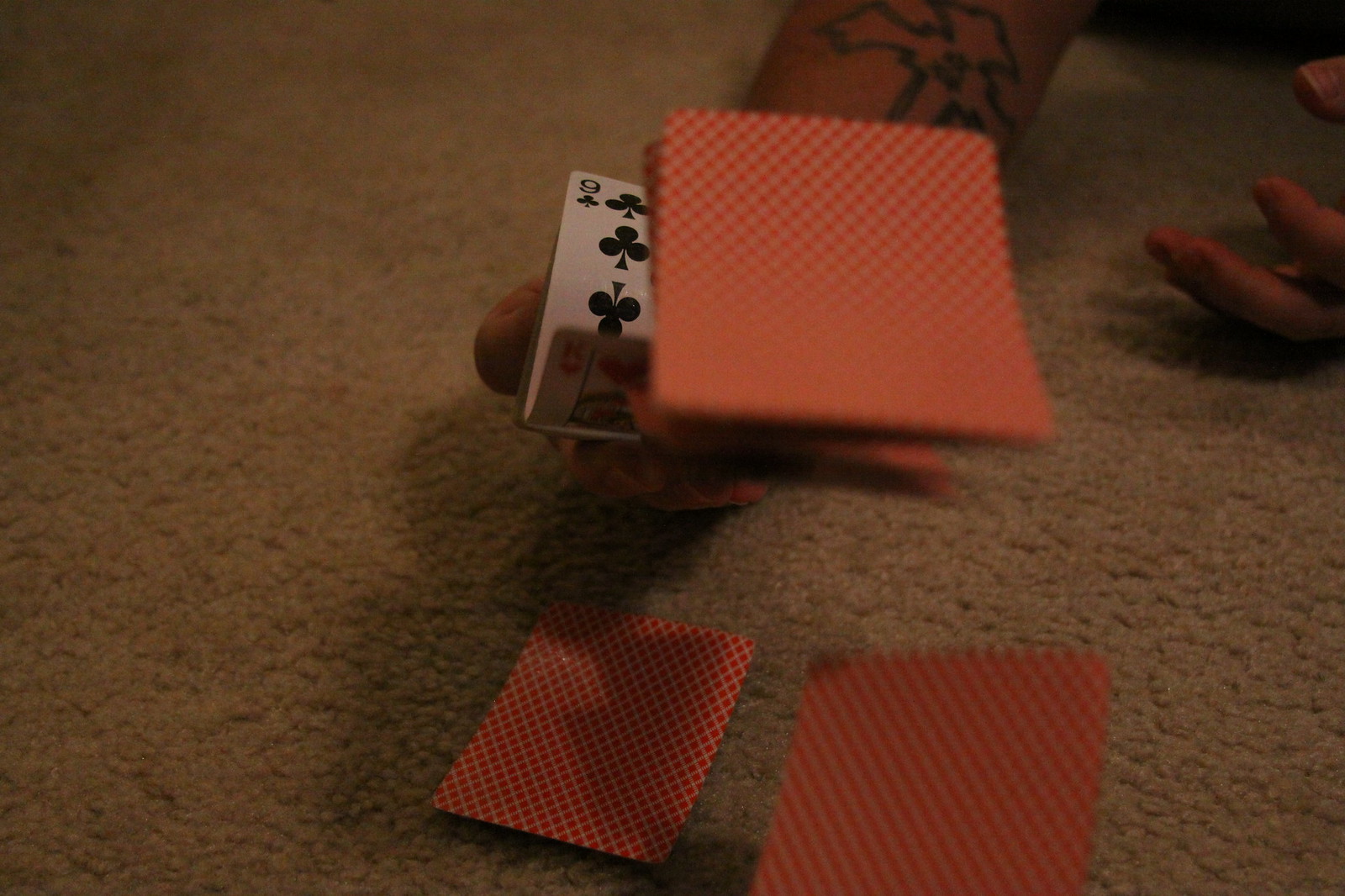In this captivating photograph, an individual deeply engaged in the art of cardistry is captured in a moment of dynamic action. The dimly lit setting accentuates the dramatic flair of the scene, where playing cards are manipulated with extraordinary skill. The focal point of the image is a flurry of playing cards, caught mid-air as they appear to spring from the top of a deck with remarkable velocity, suggesting rapid and expert handling. 

The cards, momentarily suspended in flight, are slightly out of focus, effectively conveying their swift movement. One card, however, stands out in sharp clarity on the carpeted floor—the nine of clubs—highlighting the precision involved in the performance. Surrounding this sharply focused card are others in various stages of descent, a few already scattered on the floor, creating an almost magical cascade effect.

The individual's hands, clearly skilled and steady, are central to the composition. One hand, turned upward, appears to be releasing the cards, while the other rests firmly on the soft nap of the carpet, securely holding the deck from which the cards spring. The forearm and an adjacent hand poised on the carpet imply steadfast control and provide context to the controlled chaos of cardistry in progress. 

Overall, the photo brilliantly captures the sophisticated artistry and kinetic thrill of cardistry, where precision, dexterity, and a touch of unpredictability come together in a visual dance of playing cards.